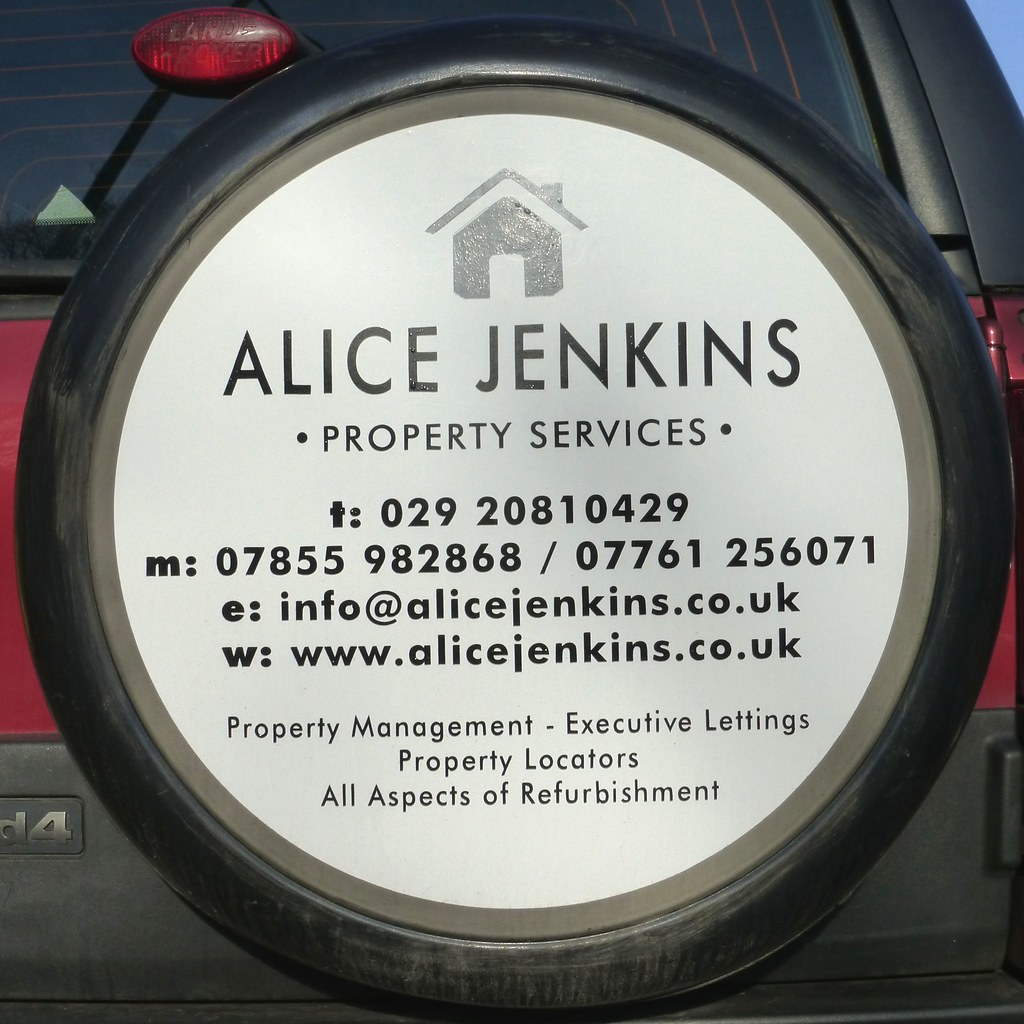The image features a close-up photograph of the back of a gray SUV, focusing on the spare tire cover, which has been utilized for an advertisement. The tire cover is predominantly white and prominently displays the name "Alice Jenkins" in black text, alongside a small house logo at the top. Beneath the name, the ad reads "Property Services," followed by contact details that include telephone numbers, an email, and a website address: alicejenkins.co.uk. The advertisement details the services offered, listing "Property Management, Executive Listings, Property Locators, and All Aspects of Refurbishment." The SUV has noticeable red taillights, a visible rear windshield, and the upper right corner of the image captures a clear blue sky, emphasizing a bright day. The ad, positioned strategically on the spare tire cover, suggests the vehicle is part of a company fleet, making the information visible when the vehicle is out in public.